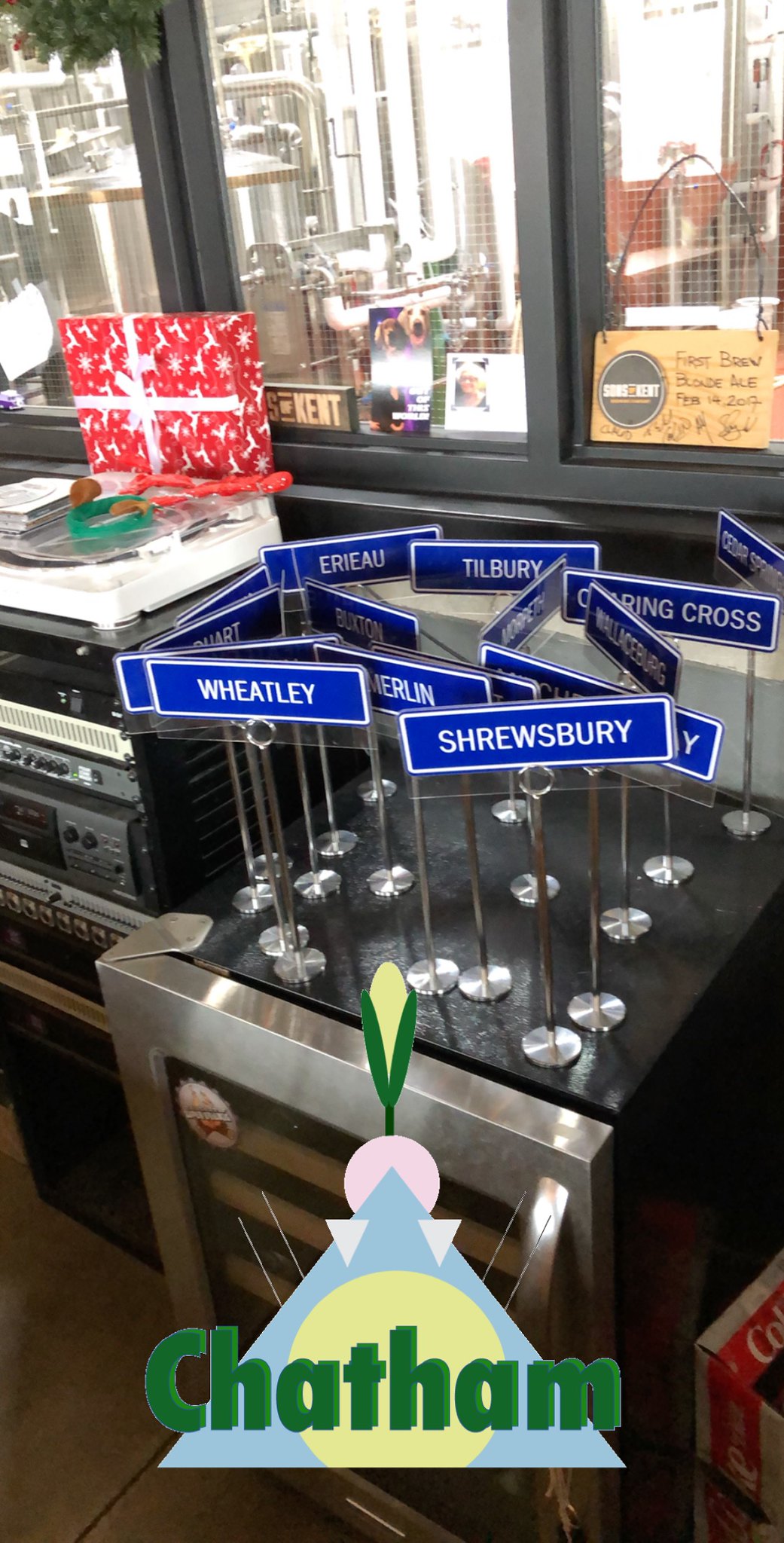The image depicts an interior scene, possibly of an office or breakroom, featuring a beverage cooler or wine fridge with gray metal atop and brown slatted doors. Stacked on top of the cooler are metal sign holders with blue signs in white all-capital letters reading "Wheatley," "Shrewsbury," "Tilbury," "Charing Cross," and "Arrow." To the left of the cooler is a setup of various audio or radio equipment. Atop this equipment sits a red box wrapped like a gift with a yellow and white ribbon. The background reveals windows offering a view of tall buildings and external signage. In the lower portion of the image, there is an overlay featuring a blue and yellow triangle with a smaller pink circle at the top, overlaid with bold green font spelling out "Chatham." The lower right corner shows a partial red Coke box, identifiable by its white "Coke" lettering.